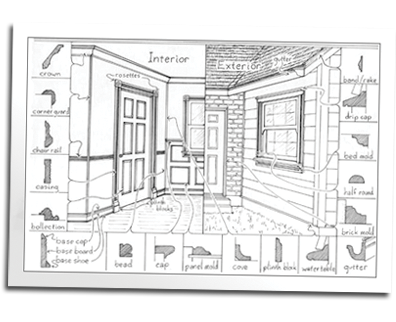This detailed architectural drawing in black and white showcases the interior and exterior design elements of a building. The central image is divided into two halves: the left side labeled "Interior" and the right side labeled "Exterior," with clear, dark text. The interior half portrays a room with a white ceiling, white walls, a door, a window, and light-colored flooring. Surrounding the central images are multiple smaller labeled sketches aligned in a U-shape around the left, right, and bottom sides, with arrows indicating specific architectural details on the central images.

The interior section highlights various types of moldings such as crown molding, baseboards, beads, caps, and corner moldings, demonstrating their placement around doors, windows, at the junction between the ceiling and wall, and possibly mid-wall where chair rails might be found. The exterior part illustrates elements like light-colored brick, siding, and a dark roof, focusing primarily on guttering systems and exterior trim around doors and windows. This drawing serves as an illustrative guide, likely intended for carpenters or architects, detailing the intricate design components and decorative features used in both interior and exterior home construction.